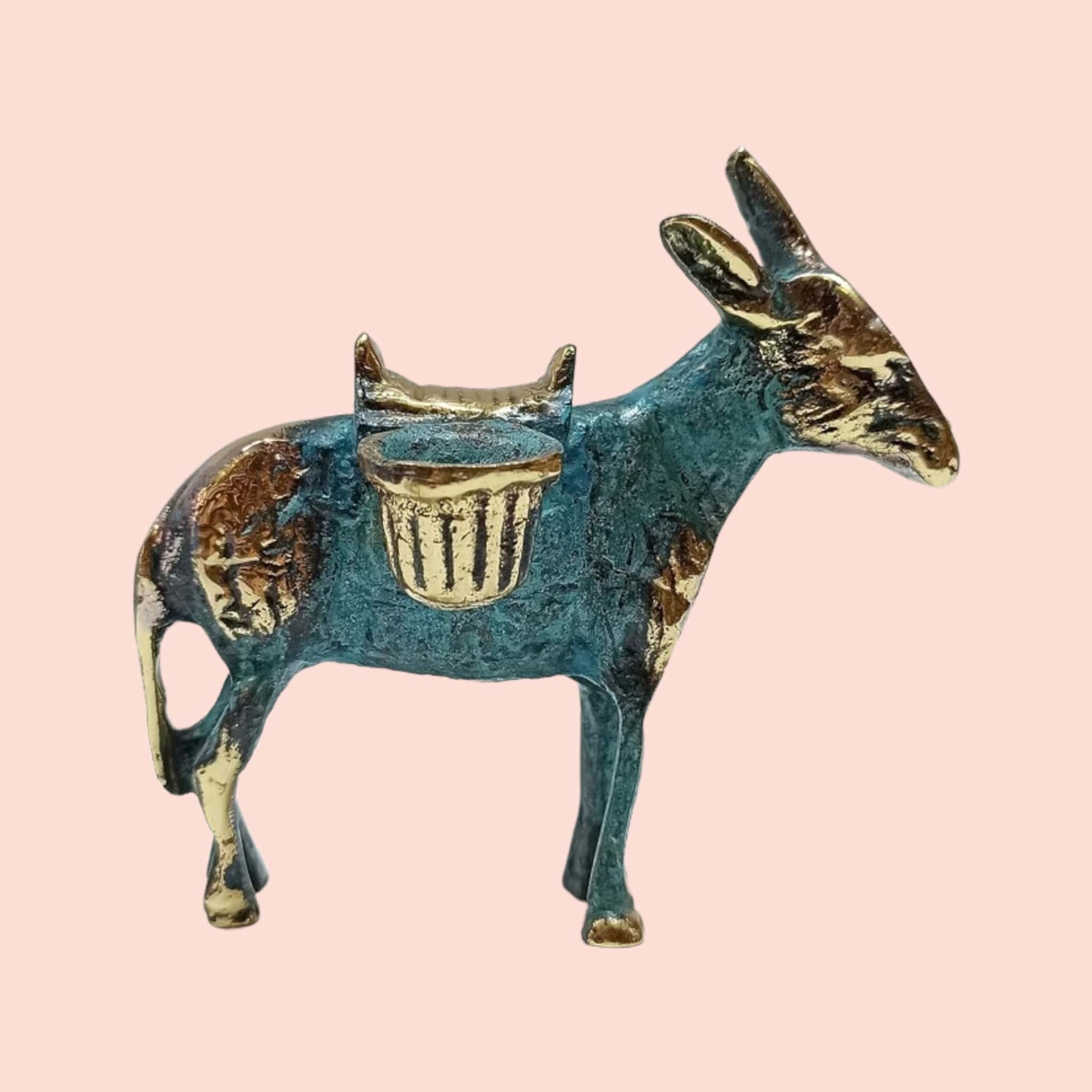The detailed photograph captures a small, intricately carved figurine of what appears to be a donkey, likely an artifact, museum display, or contemporary artwork. The donkey-shaped sculpture stands out against a solid, light peach or pink background. It features a striking combination of colors and materials: its head, saddle, and back hooves are a shiny golden color, while its body is predominantly a teal or light blue hue, possibly indicative of a metal like copper. The sculpture is adorned with gold accents, particularly around its head, ears, and back hooves, giving it a polished and reflective appearance. The statue has a long tail, a seat on its back that resembles a saddle, and a distinct pattern on its side shaped like a water basket. Despite the shiny elements, the texture of the figurine overall is gritty with multiple marks, adding to its intricate and detailed craftsmanship. The size of the sculpture seems to be small, possibly slightly larger than a cell phone, highlighting its delicate construction.